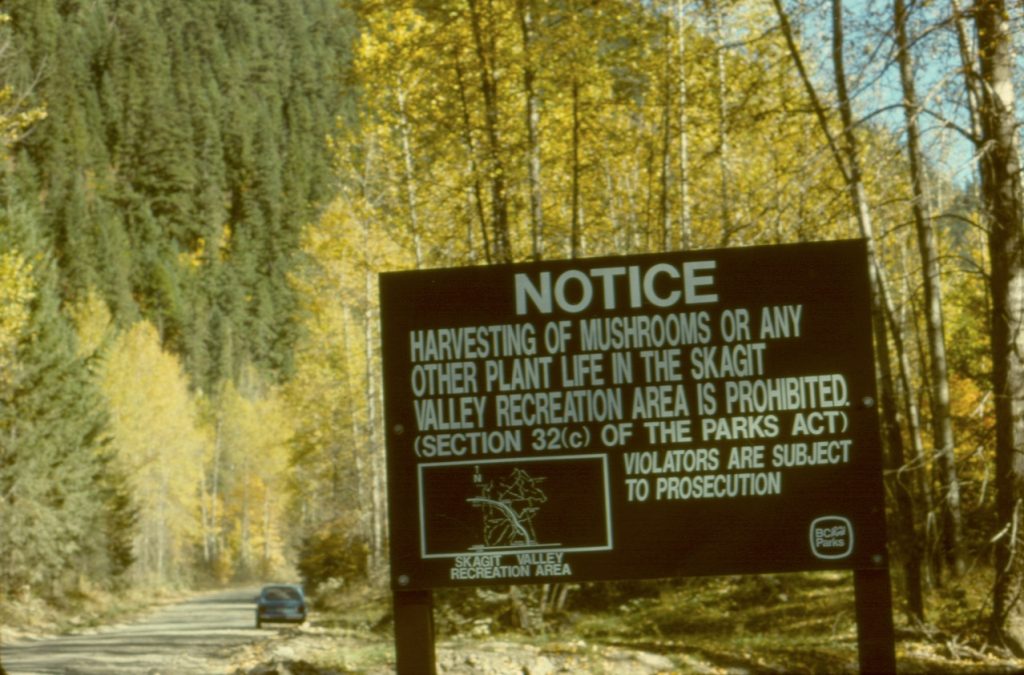This is an outdoor photograph that appears to be from the 1980s or 1990s, depicting a forested area with a sunlit dirt road, possibly unpaved. Prominently featured on the center right is a large, brown metal sign mounted on two metal poles. The sign bears a warning in white lettering: "NOTICE: Harvesting of mushrooms or any other plant life in the Skagit Valley Recreation Area is prohibited. Section 32C of the Parks Act. Violators are subject to prosecution." At the bottom left of the sign, there is a small map labeled "Skagit Valley Recreation Area" with a line indicating the trail or road's path. A blue car is parked on the dirt road to the left of the sign. The backdrop includes several trees with varying shades of green foliage, some exhibiting hints of yellow, suggesting seasonal change. The forest canopy allows sunlight to filter through, illuminating parts of the road and highlighting the blended colors of the tree leaves. Above in the upper right corner, a clear blue sky is visible, enhancing the serene, natural atmosphere of the scene.